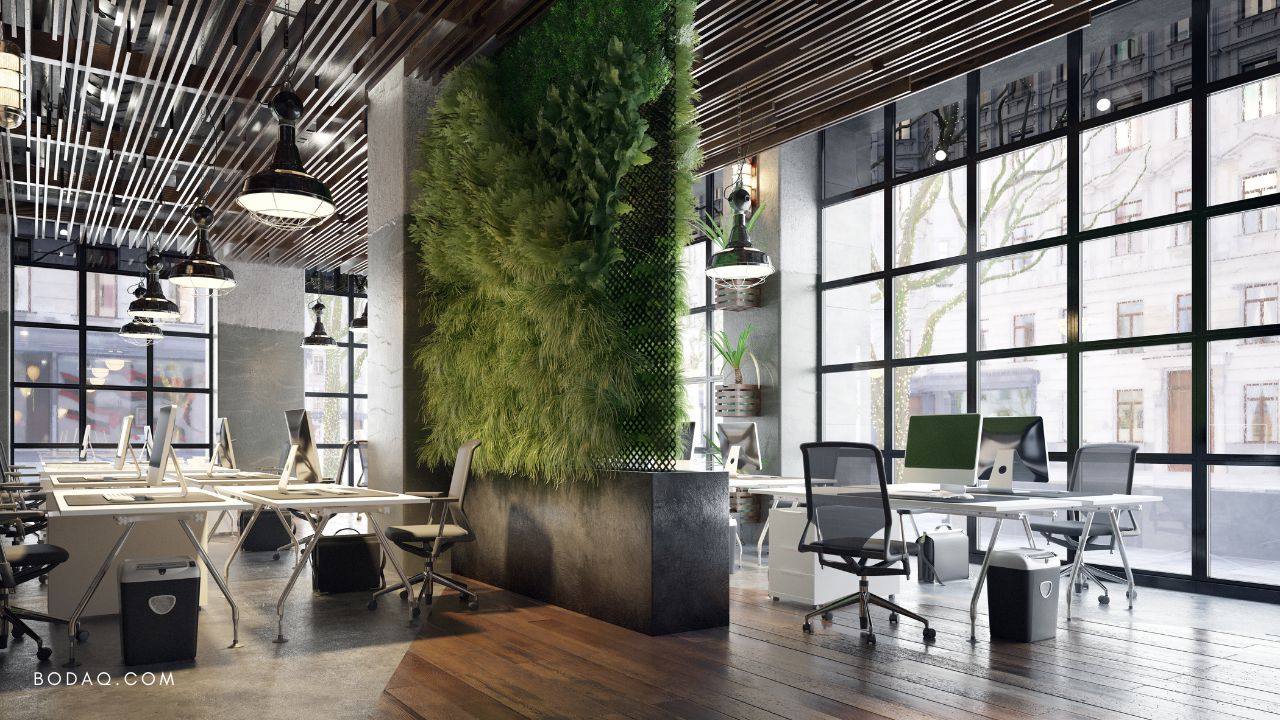The image depicts a bustling, urban office loft with a modern and industrial aesthetic. The spacious interior is furnished with numerous white desks, each paired with industrial-style office chairs and equipped with personal computers, primarily Macintosh models. The loft, part of an eye-catching Bodak (bodaq.com) workspace, features a combination of hardwood floors and other types of flooring. Distinctive black, industrial lamps hang from the ceiling, striking a balance between the abundance of natural light streaming through the large, tic-tac-toe pattern windows on the sides and front of the building, and the artificial illumination within.

In addition to the computers, each workstation is equipped with either shredders or trash cans, ensuring a well-organized and functional environment. The office is situated in a bustling city area, characterized by various architectural styles and tree-lined streets, adding to its dynamic ambiance. The setting appears to capture a winter scene, as inferred from the subdued sunlight and the indoor lights being actively used despite the daytime. Overall, this work loft exemplifies a contemporary and efficient workspace designed for productivity and collaboration.